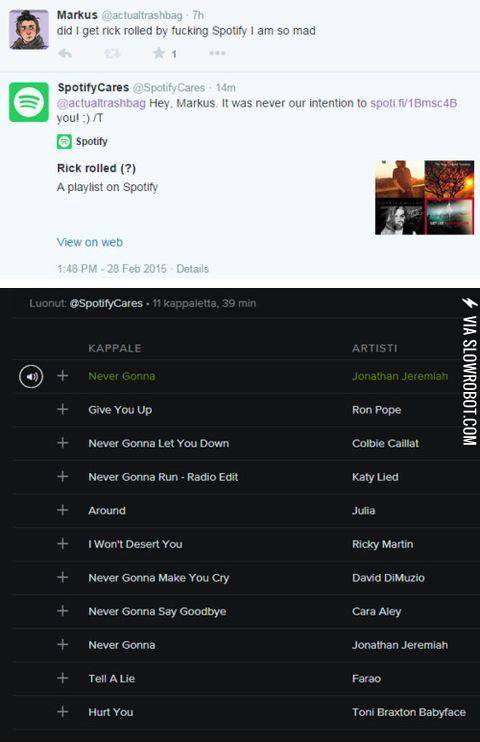The image is a portrait-oriented screenshot of a comment thread and Spotify playlist interaction. The aspect ratio indicates the photo is about twice as tall as it is wide. The upper part of the image has a gray background, while the lower part transitions to a black background.

At the top of the image, there is an avatar of a man with a topknot, named Markus (spelled M-A-R-K-U-S). Next to his avatar, it says "@ActualTrashBag - 7 hours ago". His comment reads: "Did I get Rickrolled by fucking Spotify? I am so mad."

Below Markus's comment, there is a response from Spotify, identified by a green icon with a white center that says "Spotify Cares". Their comment reads: "Hey Markus, it was never our intention to", followed by a hyperlink, which seems to lead to a page titled "Rickrolled? A playlist on Spotify". Below the hyperlink, the incomplete playlist is shown, listing four album titles.

Further down, against a black background with white text, there's a continuation of the conversation, again from "Spotify Cares". This part shows a playlist named "Rickrolled? - 39 minutes ago". The playlist is creatively arranged to mimic the lyrics of Rick Astley's song "Never Gonna Give You Up". Each song title sequentially forms the lyrics of the song. The titles listed include:
- "Never Gonna" by Jonathan Jeremiah
- "Give You Up" by I'm Hope

The playlist continues in this fashion, with each song title following the lyric sequence of the famous Rick Astley tune, making it a cleverly constructed Rickroll.